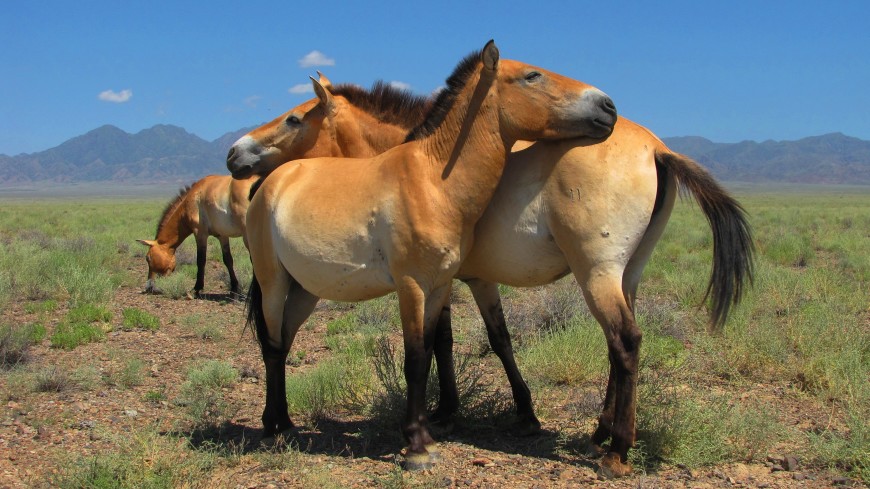In a wide, open field dotted with green patches, brown dirt, and occasional rocks, stands a peaceful scene of three equines—two horses or mules, and one in the background likely a horse or mule. The foreground showcases two light brown and white animals standing side by side but facing in opposite directions, their dark brown manes and tails cascading down from their bodies. Their legs fade into a dark brown, almost black hue, grounding them in the rocky, earthy terrain. Slightly behind them on the left, another similarly colored animal bends down to graze on the grassy patches. In the distance, majestic, barren mountains form a stark contrast against the bright, turquoise sky, which is interspersed with a few white clouds. The scene conveys a sense of tranquility and familiarity among the animals, comfortably nestled and relaxed under the open sky, indicative of a sunny day even though the sun itself is not visible.